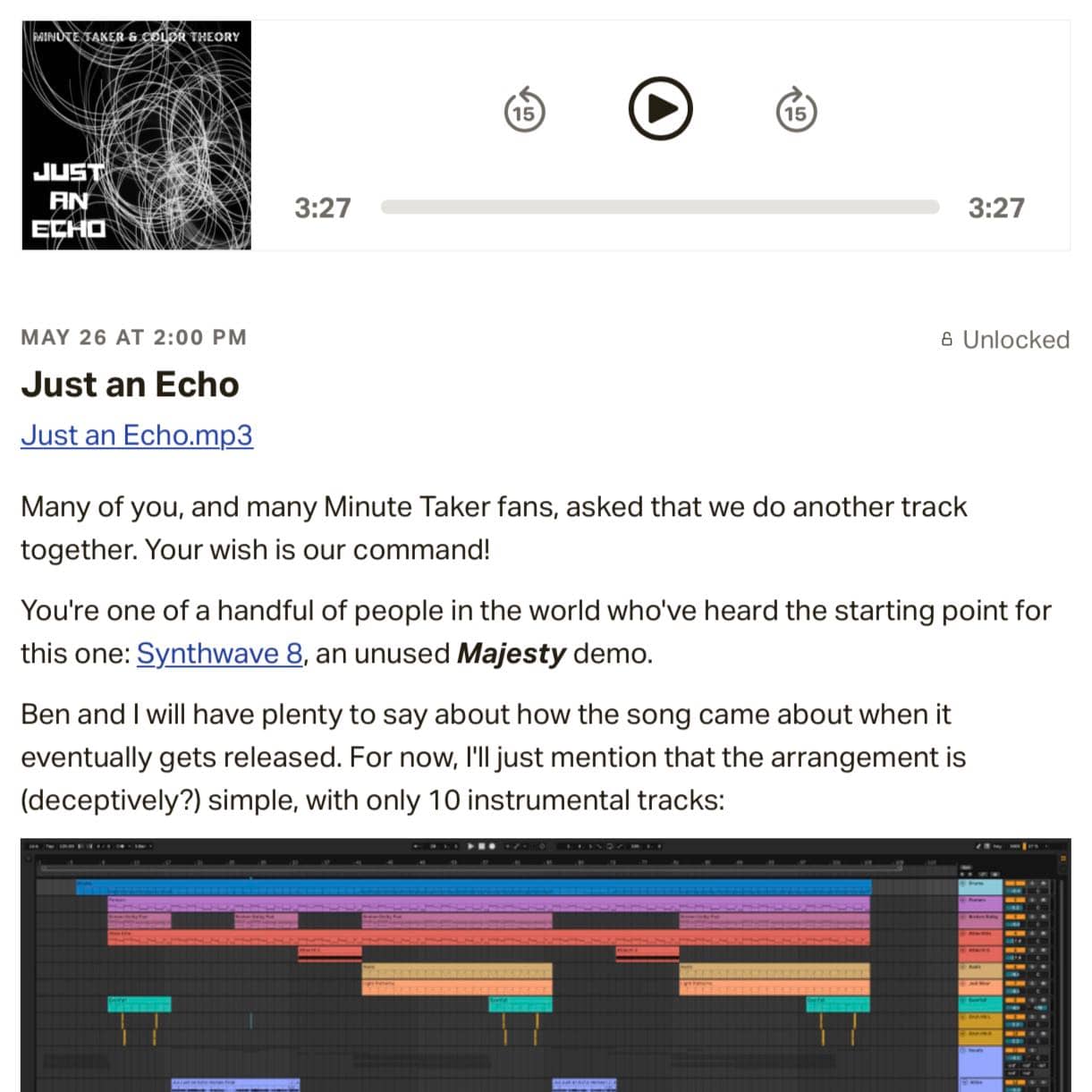The image depicts a music player interface with a minimalist black box and white curvy lines, displaying the title "Just an Echo." Prominent buttons include a play button, and 15-second skip buttons for both backward and forward navigation. The status bar indicates a duration of 3 minutes and 27 seconds.

Below this, the date and time "May 26th at 2 PM," is displayed alongside the track title "Just an Echo" again. Beneath this, an underlined blue text reads "just an echo.mp3," suggesting it is a clickable link.

In the upper right corner of the image, there is an "Unlock" button. Further text in the image reads: "Many of you and many Minutetaker fans asked that we do another track together. Your wish is our command. You're one of a handful of people in the world who heard the starting point for this one." This is followed by another blue underlined text: "Synthwave 8," labeled as "an unused magistrate demo."

The message continues, "Ben and I will have plenty to say about how the song came about when it eventually gets released. For now, I'll just mention that the arrangement is deceptively simple with only 10 instrumental tracks." 

Below this text, the image shows a screenshot of Pro Tools or other music production software, featuring several colorful horizontal bars representing different instrumental tracks aligned from left to right.